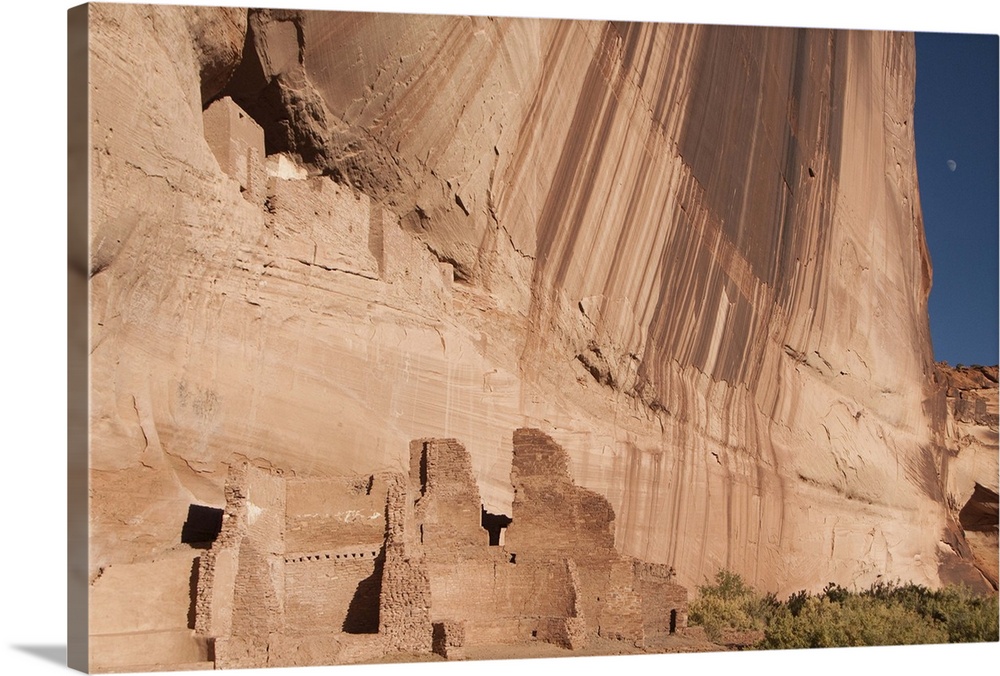The image is a color photograph captured in an outdoor desert setting, taken just before nighttime. The scene is dominated by a massive rock formation that spans most of the area, featuring various shades of brown with long, vertical streaks that suggest recent wetness. The rock formation, similar in essence to those found in the Grand Canyon region, has a rugged and intricate texture. The ruins of an ancient village, built from stone or brick that blends seamlessly with the mountainous backdrop, are nestled into the side of this colossal structure. Sharp, jutting rocks are visible in the foreground, punctuating the landscape with dramatic edges. At the bottom right, sparse vegetation, including a small grassy patch and some foliage, adds a touch of green to the earthy tones of the scene. The sky, a serene blue, reveals half of a dim, white moon, providing a gentle celestial touch in the background.